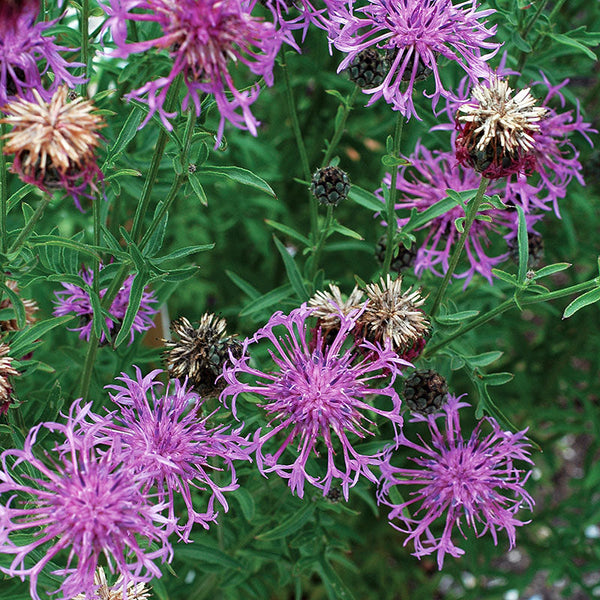This image showcases what appears to be an AI-generated visual of purple flowers captured with a phone or regular camera. The flowers possess uniquely odd and intricate structures, with each one having a central spherical bud from which multiple purple shoots extend. There are approximately ten such purple flowers arranged throughout the frame, each resembling a spider with its petals arching out and fanning open at the ends. Among these vibrant blooms, there are also five cream-colored flowers, suggesting either dried or wilting stages. Surrounding this colorful display, very lush and deep green plants grow densely, resembling the unrestrained spread of weeds, yet indicative of an actual planned garden. Scattered among the flowers are small bulb-like formations, reminiscent of blackberries with their clustered, spherical shapes. The background is slightly blurred due to a high depth of field, adding to the picture's depth and focus on the foreground blooms, which themselves are captured with remarkable clarity and richness in detail.